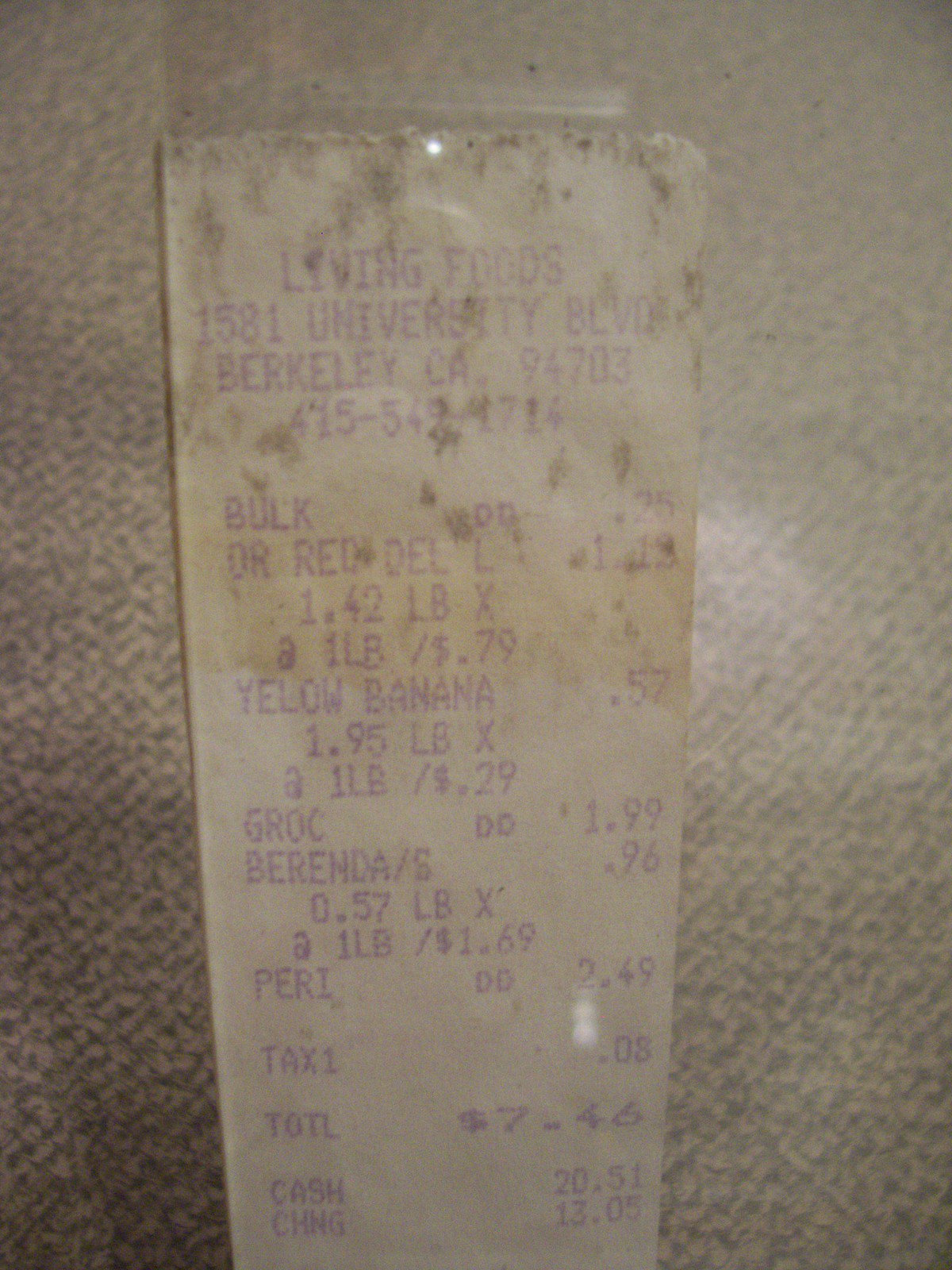The image features an old, stained receipt from Living Foods, located at 1581 University Boulevard, Berkeley, California, 94703. The receipt is notably dirty on the upper half, with possible signs of mold or grease stains. The text and print on the white receipt are in a light purple or blue hue. 

From the top, the receipt details the store's name and address, followed by a phone number, 415-549-4714. The purchased items include: "DR Red DELL," "Yellow Banana" priced at $0.57 and $1.95 per pound, "Groceries" at $1.99, "Berendas" at $0.96 and $0.57 per pound, and "Perishables DD" at $2.49. The item costs and quantities, along with their respective prices per pound, are listed on the right. 

Towards the bottom, the receipt outlines the tax paid, totaling $7.46. The amount tendered was $20.51, resulting in a change of $13.05. The overall condition of the receipt suggests considerable age, with noticeable splotches and dinginess contributing to its worn appearance.